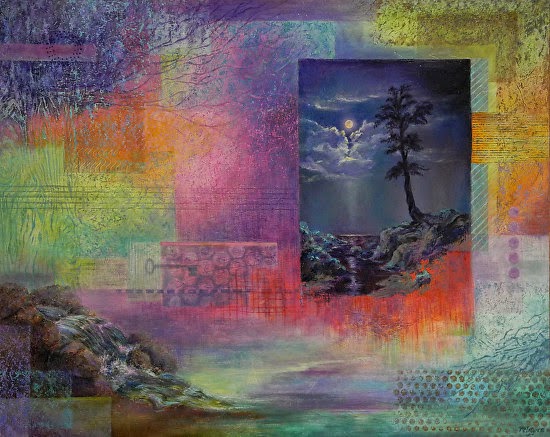This captivating, computer-generated image effortlessly combines elements of a painting and graphic art, presenting an intricate and colorful scene. Dominating the right-hand side is a detailed portrayal of the night sky, featuring a luminous full moon peeking through soft clouds. Beneath the celestial display, a tree emerges prominently from a small hill, its branches reaching upwards, set against a backdrop of shimmering water. 

In the center of the composition, a prominent vertical rectangle showcases a vivid nighttime landscape where the moonlight bathes a solitary tree and a rugged mountain range in a serene glow. Surrounding this central scene, a diverse collage of colors—purple, pink, green, orange, yellow, blue, and red—expertly blend together, creating a vibrant and dynamic atmosphere.

The bottom left and right of the image depict water flowing gracefully across the scene, enhancing the sense of movement and continuity. Additionally, a smattering of dots adds texture and depth throughout the artwork. The intricate array of branches, leaves, unique areas, and varied shapes contribute to the richness and complexity of the piece, making it a visually arresting masterpiece.